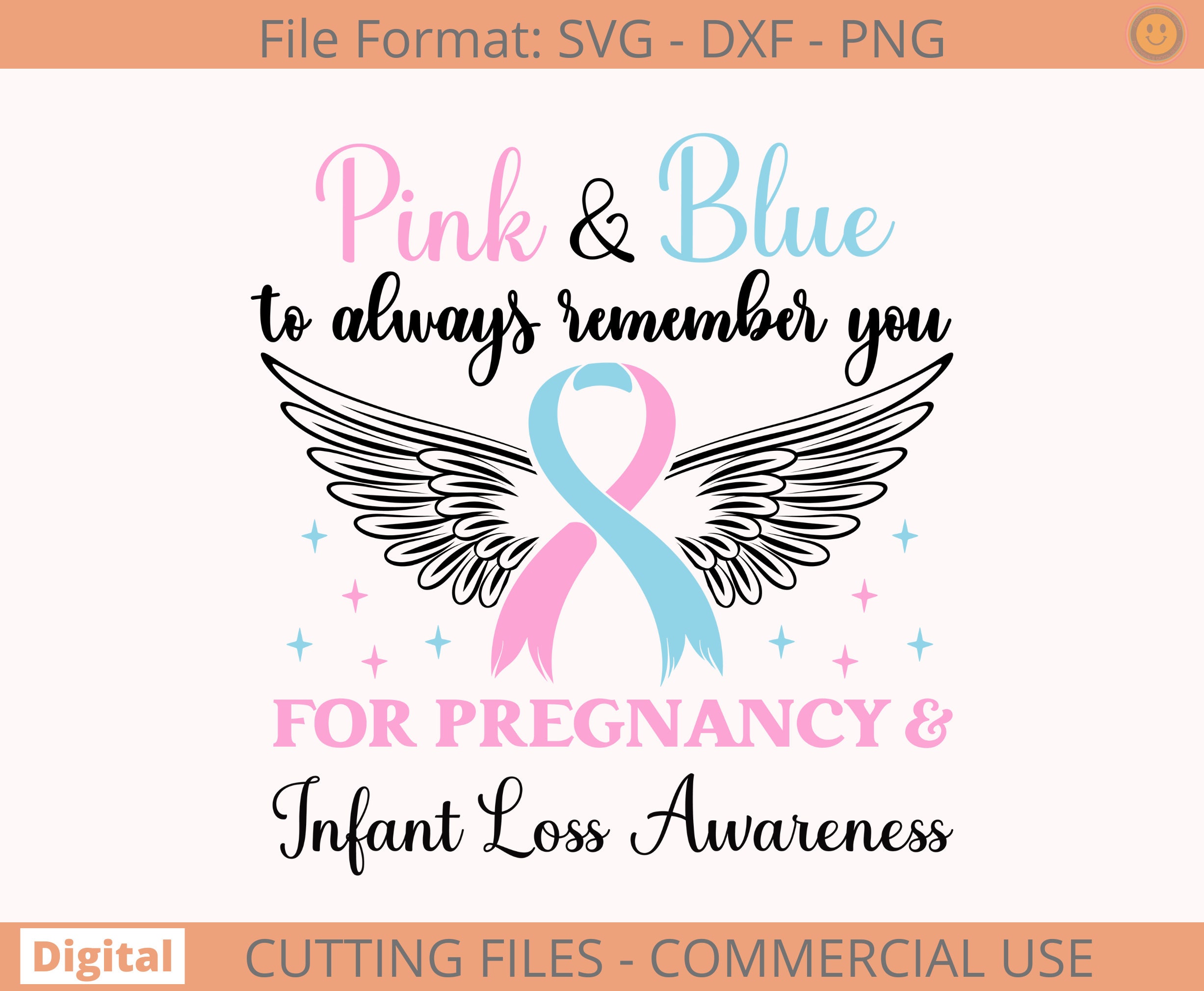The image is an advertisement for Pregnancy and Infant Loss Awareness. It features a crossed ribbon in light blue and pink, representing boys and girls, with angel wings behind it and scattered stars in blue and pink. The text at the top of the image reads "pink and blue" in matching colors, followed by "to always remember you" in black cursive. Below the ribbon, it says "for Pregnancy and Infant Loss Awareness" with "for Pregnancy" in pink and "and Infant Loss Awareness" in black cursive.

The entire advertisement is presented on a white background with an orange border at the top and bottom. At the top of the image, grey text reads "File Format SVG DXF PNG," alongside a light orange smiley face with a grey border. At the bottom, an orange block contains bold orange text reading "digital cutting files" and grey text on the right that says "- commercial use".